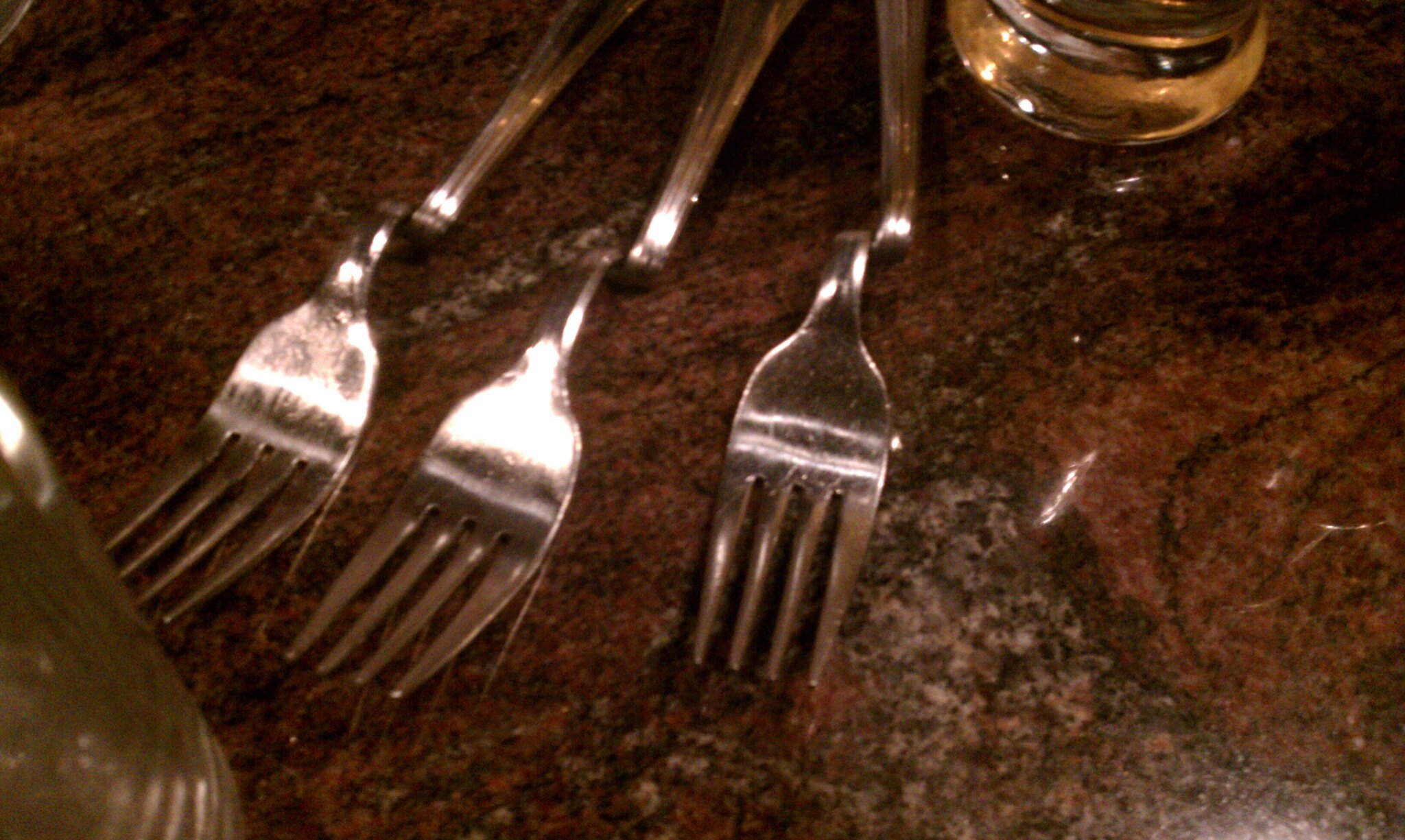The image features three silver forks, each with four prongs, lying on a maroon, gray, and white granite countertop. The forks are aligned side by side, though not perfectly parallel, and they lean slightly to the left. An eccentric, sharp bend is present just above the pronged heads of each fork, causing their handles to twist and curve back, as if broken but still attached. Bright white light reflects off the two forks on the left, while the one on the right shows some speckled reflections. In the bottom left corner of the image, there is a foggy glass bottle, and in the top right corner, a short glass container filled with yellow liquid. The scene also includes a shiny gold mug with a black ring around the top, adding extra detail to the countertop's diverse texture and color palette.